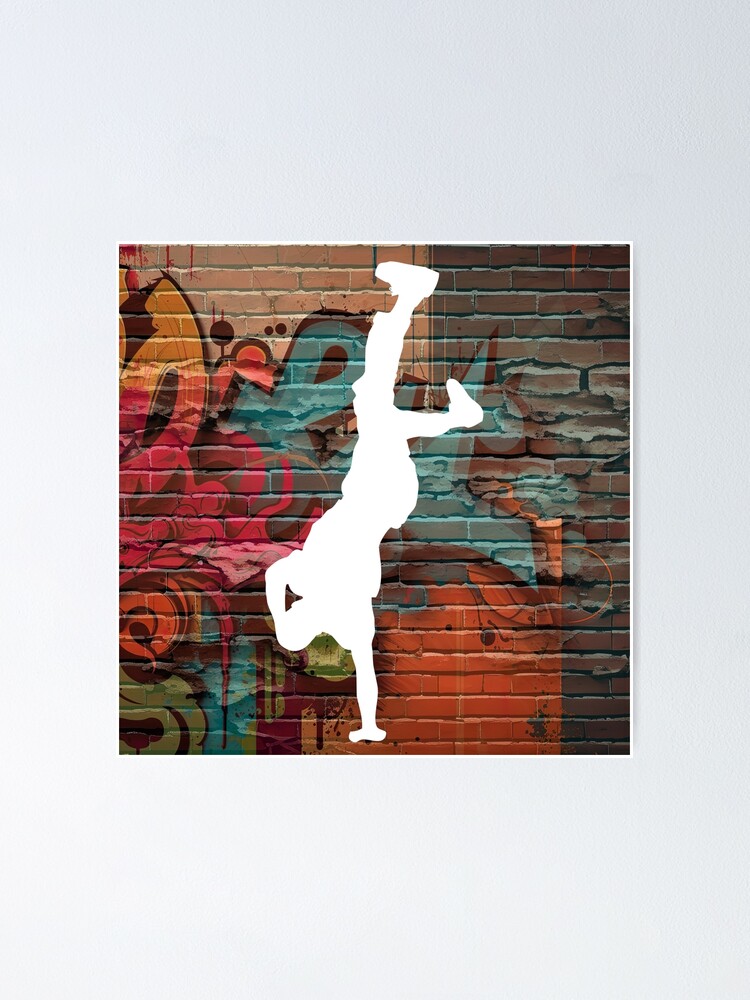The image presented is a visually captivating poster set against a vibrant graffiti-adorned brick wall. The mural showcases a mix of colors, predominantly shades of orange, red, brown, and light blue, creating a dynamic urban backdrop. At the center of the composition, a strikingly solid white silhouette of a breakdancer captures attention. This dancer is impressively balanced on one hand, with the other arm touching their head. One leg extends straight up, while the other is bent, emphasizing the fluidity and strength of the pose. On the lower right-hand corner, the red brick wall is partially visible, while the left side of the background features stylized flowers and petals in hues of red and pink, along with blue accents interwoven in the graffiti. This detailed and vibrant poster beautifully melds the art of breakdancing with the energetic essence of street art.